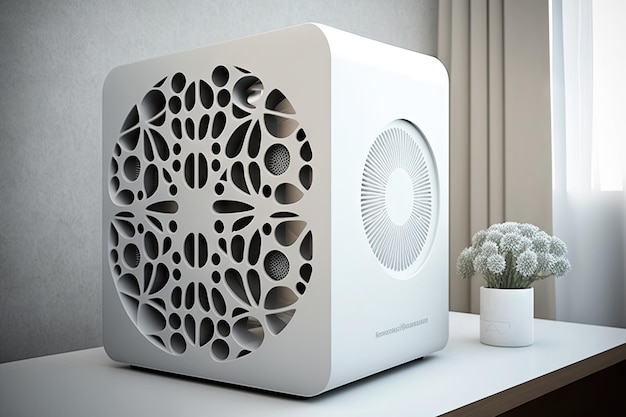In a serene setting marked by minimalist decor, a distinctive white cube sits prominently on a white tabletop. This cube, which could plausibly be a sophisticated speaker or humidifier, features intricate etchings and holes in the form of teardrops, circles, and semi-circles. The cube boasts a detailed front panel with a circular pattern made up of thin, round fins surrounding a central cap. A subtle logo adorns this panel, though its specifics are not easily discernible. The scene is bathed in natural light streaming through a window, flanked by curtains, which casts a soft glow against a gray wall. Adjacent to the cube is a small white pot containing green stems topped with spiked white and green ball-like flowers, adding a touch of nature to the contemporary tableau.